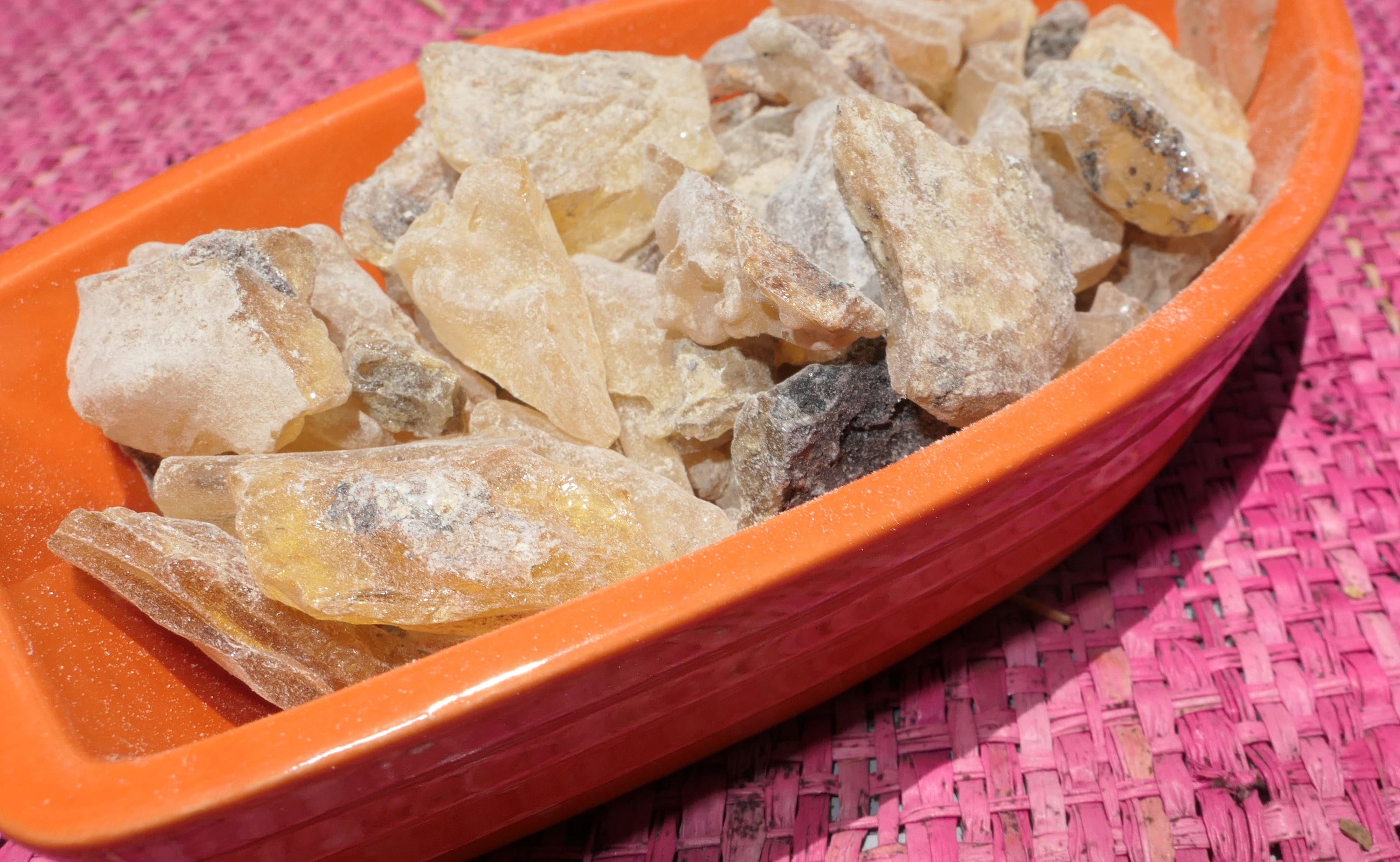The image features a vivid pink woven mat serving as a backdrop for a striking, boat-shaped orange ceramic bowl. Inside the bowl, a collection of various crystals or stones is prominently displayed, with each piece contributing to an array of colors and textures. The bowl features around 10 to 15 stones, which range in color from bright citrine yellow to dark charcoal gray, with occasional hues of ashy white, tan, and even hints of orange. The surfaces of these stones appear dry and powdery, leaving a visible residue on the interior and rim of the bowl. Some stones have cracked areas revealing smoother, shinier surfaces. The stones are all of similar size and are neatly stacked within the long, boat-like orange container, enhancing the vibrant and detailed composition of natural elements against the colorful mat.